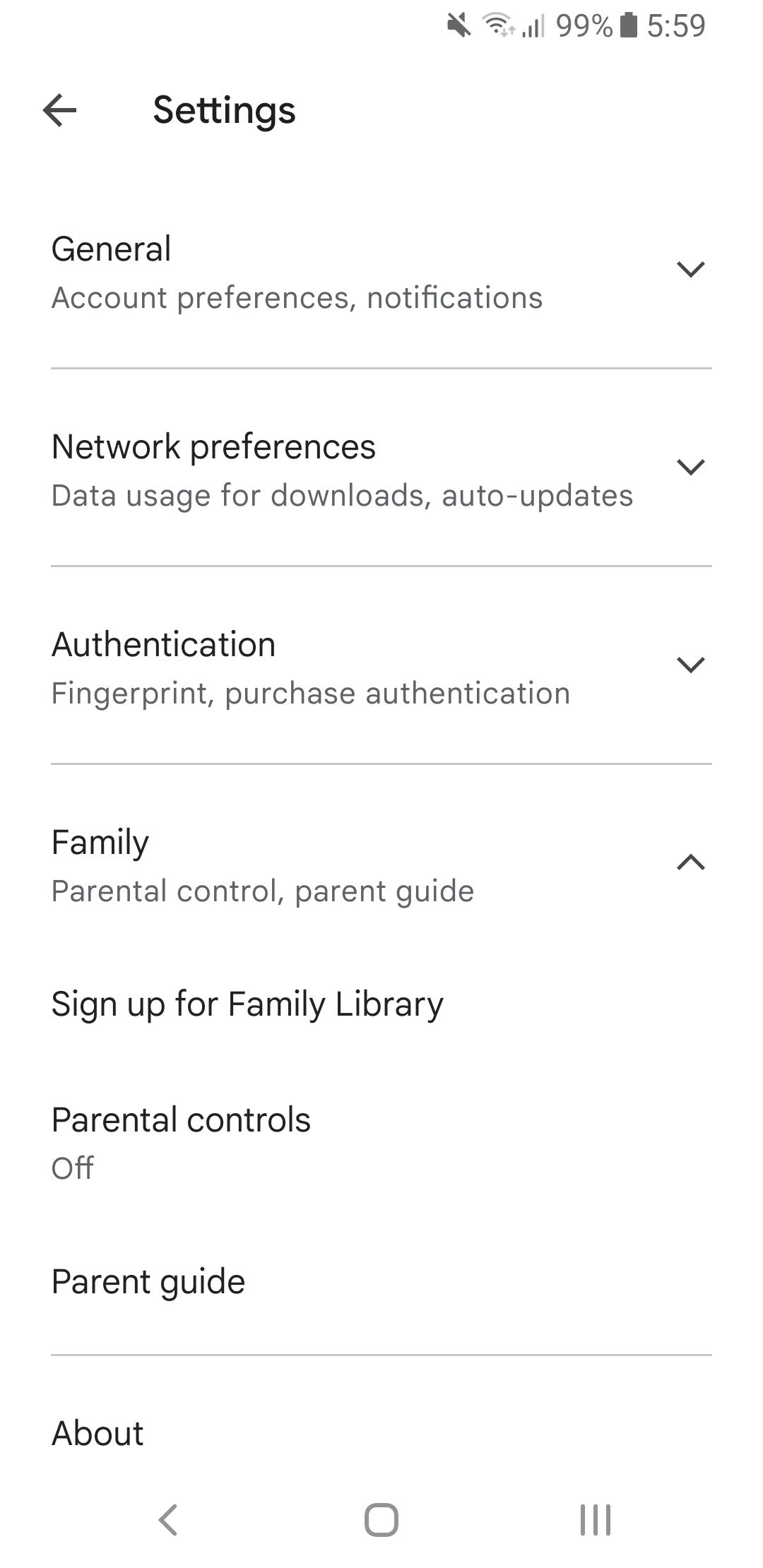This image features a screenshot of an Android device's interface. In the top right corner of the screen, the status bar displays essential indicators: the battery level is at 99%, the time is 5:59, the Wi-Fi signal strength icon is visible, and the network signal bar is present. 

The central portion of the screenshot shows a list of menu options, suggesting that the user is likely within a settings or preferences section of an application. The visible texts include:
- Settings
- General
- Account Preferences
- Notifications
- Network Preferences
- Data Usage for Downloads
- Auto-Updates
- Authentication
- Fingerprints
- Purchase Authentication
- Parental Controls
- Parental Guide
- Family
- Sign up for Family Library
- About

At the bottom of the screen, the familiar Android navigation keys are displayed, including the back button, the home button, and the recent apps button. These details collectively indicate that the screenshot is taken from a settings menu related to account and device management on an Android device.